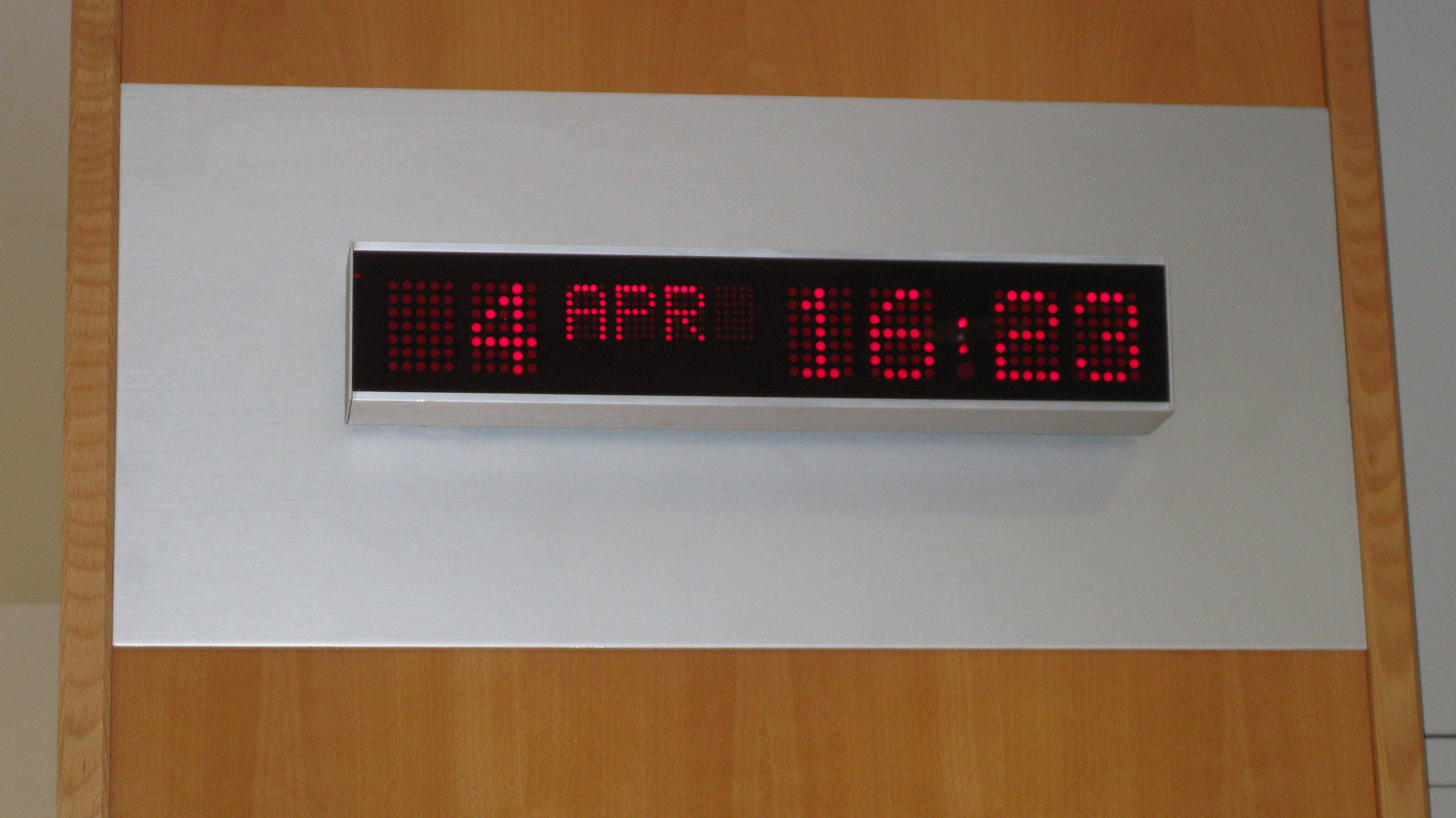A digital clock is prominently mounted on a light wooden-colored door, displaying both the date and time in striking red LED digits. The clock's frame is white, giving it a clean and modern appearance that fits seamlessly against the door. The digital display showcases "4 APR" for April 4th and "1623," or 4:23 PM, in a bold marquee style, making it easily readable from a distance. The door, likely situated in a public place, is flanked by white walls, suggesting a well-maintained and bright environment.